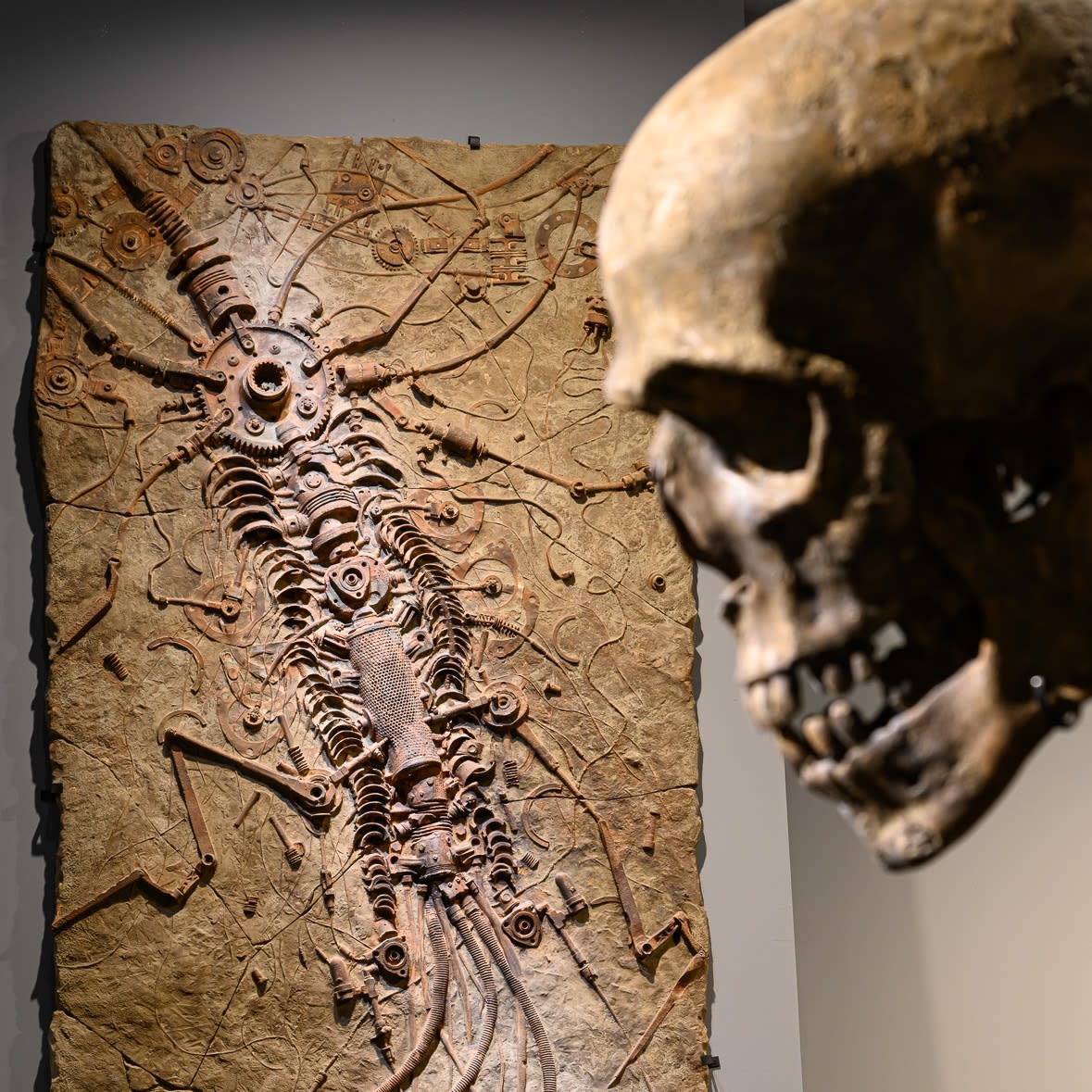The image depicts a beige-colored stone panel that appears to showcase a fossil of a futuristic, steampunk-like creature. The creature, seemingly artificial, features metallic elements such as a screw-like head, metal rod legs, gears, and ratchets, suggesting a fusion of biological and mechanical components. The background is a light gray wall, lending the scene a museum-like ambiance. 

In the foreground, there is a side view of an old, brownish skull with hollowed-out eye sockets and several missing teeth, some of which are black and decaying. The skull, jutting out from the top right corner, adds a haunting contrast to the scene with its eerie reminder of death. The juxtaposition of the mechanical "fossil" and the human skull creates a surreal and unsettling display, evoking thoughts of a post-apocalyptic or speculative future.